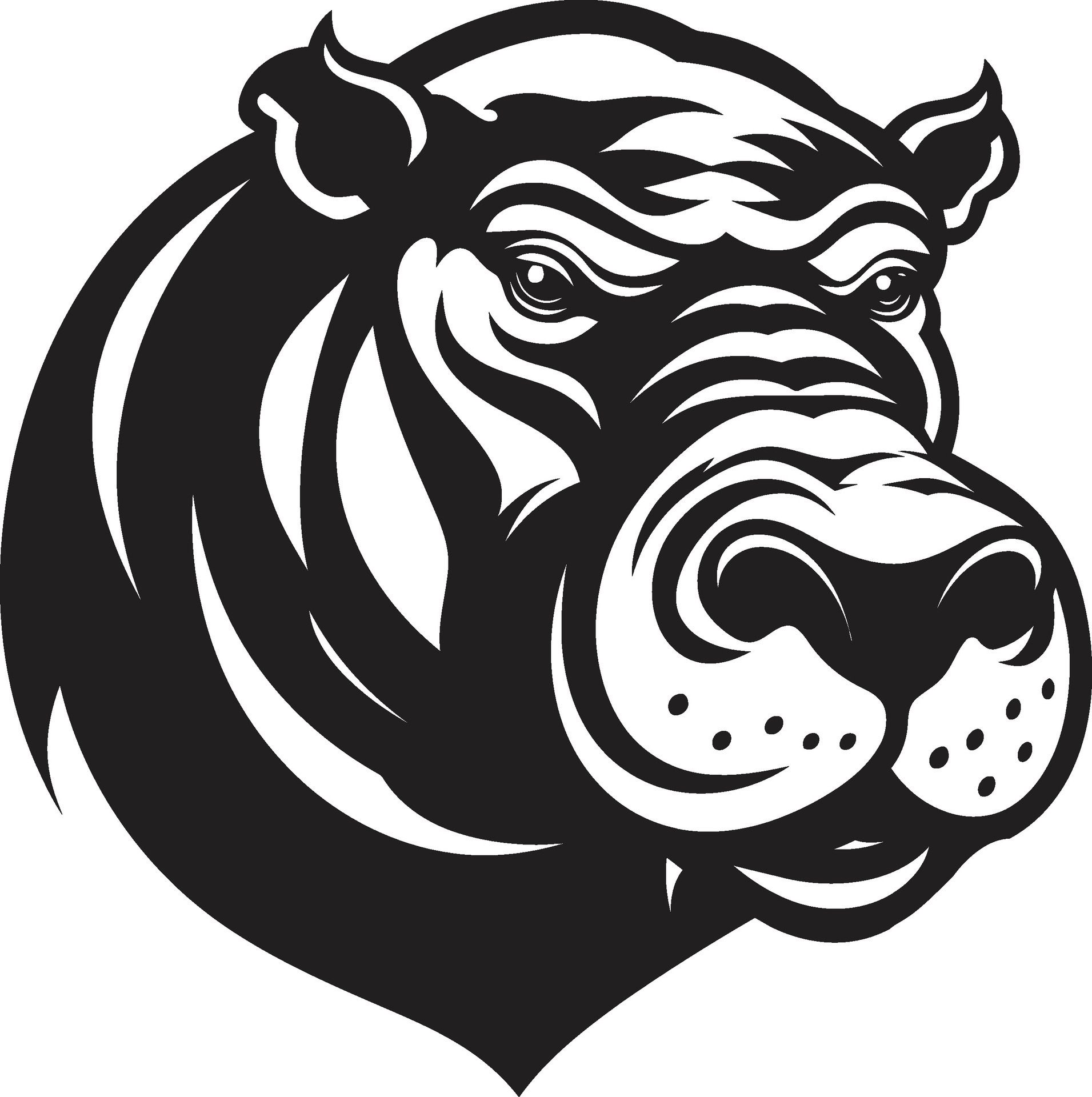This is a meticulously crafted, computer-generated black and white image of an animal's head, designed with a clipart or logo style. The heavy black outline and contrasting white inner space create striking detail and depth. The animal bears a resemblance to a hippo but also exhibits features reminiscent of a dog, bear, and lion, with a snarl suggestive of aggression, dots symbolizing whiskers on its snout, and a possible mane. Some interpretations liken it to a warthog, considering the widely-set eyes and pronounced nostrils, though notable tusks are absent. The neck is depicted with thicker lines that thin towards the snout, and the pointed ears stand upright with entirely black interiors. The image shows more of the right side of the face, maintaining a neutral expression. This stylistic portrayal, potentially created with charcoal-like strokes, is distinctly rendered in black bands that define spaces and textures, making it suitable for use as a sticker, t-shirt graphic, or logo.